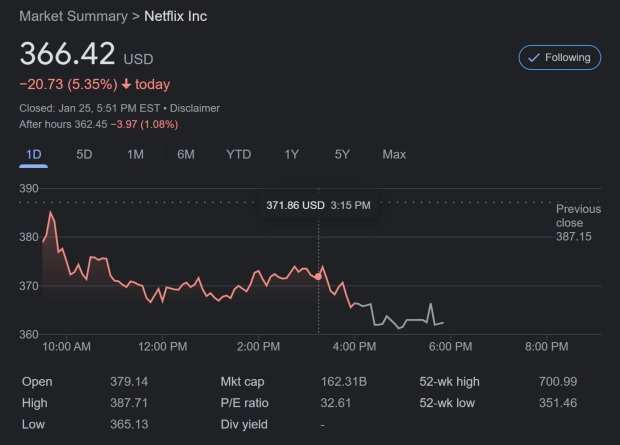This detailed screenshot captures the market summary for Netflix Incorporated. At the top, the current value of Netflix’s stock is prominently displayed at $366.42 USD. Next to this, in red text, it indicates a decline of -20.73 points, signifying a 5.35% drop for the day. The status reads "Closed January 25th, 5:51 p.m. Eastern Standard Time," with a disclaimer noting the after-hours value of $362.45, which is a further reduction of -3.97 points or -1.08%.

Beneath this section, there are clickable options for 'One Day,' 'Five Days,' 'One Month,' 'Six Months,' 'Year-to-Date (YTD),' 'One Year,' 'Five Years,' and 'Max' to allow users to view the market summary over various time periods. Currently, the time frame is set to 'One Day.' The accompanying graph illustrates a downward trend in red, tracking Netflix’s stock performance throughout the day. 

A dotted line marks the current position on the graph, indicating points that can be hovered over for more detailed information at specific times. Along the horizontal axis of the graph, time intervals are denoted, while the vertical axis lists the stock’s value in USD. Below the graph, key metrics such as the 'Open,' 'High,' 'Low,' and other significant values for the day are provided, offering a comprehensive summary of Netflix Inc.'s market performance at a glance.